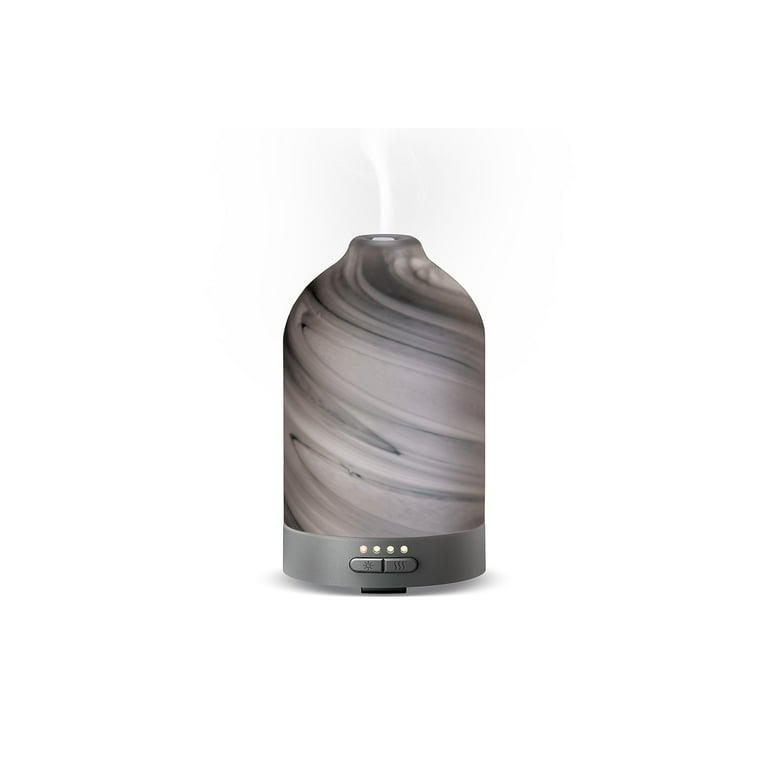This image showcases a mock-up of an automated air freshener designed to resemble a humidifier, featuring a sleek cylindrical shape that tapers into a small opening at the top from which white mist or steam appears to be emanating. The main body of the device has a sophisticated gray marble or stone swirl pattern, giving it a distinguished, natural look. It is mounted on a chrome-like base, which houses two large, adjacent buttons. The button on the left functions as the power button, while the one on the right controls the mist strength, offering four levels of intensity. Above these buttons, four yellow indicator lights are illuminated, signaling the device's current settings. The image does not contain any text, focusing purely on the visual and functional aspects of the product.